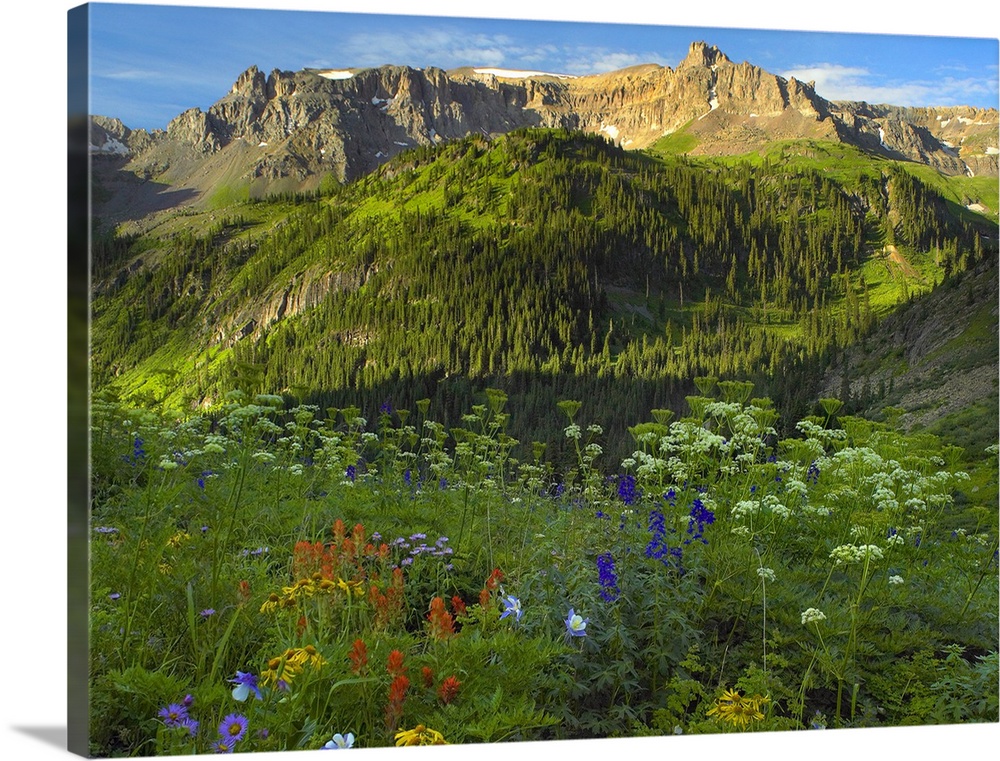The image depicts a vibrant, three-dimensional landscape of a flower-filled meadow leading to a distant forest and majestic mountains under a bright blue sky. In the foreground, an array of wildflowers in hues of purple, blue, red, yellow, and white are nestled amidst lush green grass. The flowers create a colorful tapestry that transitions into a distant forest, bathed in sunlight, with darker green trees contrasting against the surrounding grass. Further back, gray mountains topped with patches of white snow rise majestically against the sky, which is dotted with a few scattered white clouds. The entire scene is presented on a canvas that appears slightly tilted, with the left side pushed forward, hinting at its three-dimensional nature and casting a subtle shadow. The image captures the essence of a bright and sunny day, evoking the warmth and freshness of spring or summer.